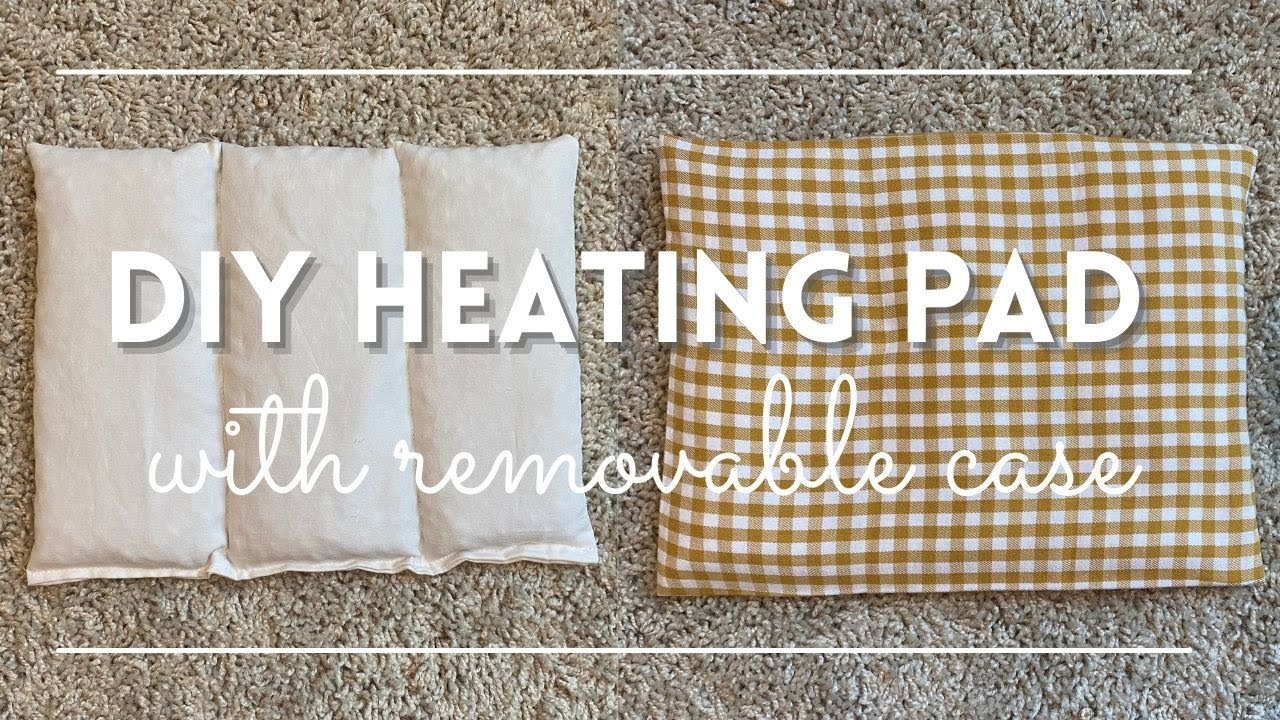The image showcases an advertisement for a DIY heating pad with a removable case. The background features a carpet that transitions from a beige hue on the left side to a gray tone on the right. Across the center of the image, a raised, bold text in white reads "DIY HEATING PAD," with a thin cursive line below stating "with removable case." On the left-hand side of the image sits a gray cushion composed of three rectangular sections sewn together. On the right-hand side is a stylish checkerboard-patterned cushion in orange and white, with alternating stripes and squares. Both items rest on the carpet, framed by a thin white line running horizontally across the top and bottom of the image.